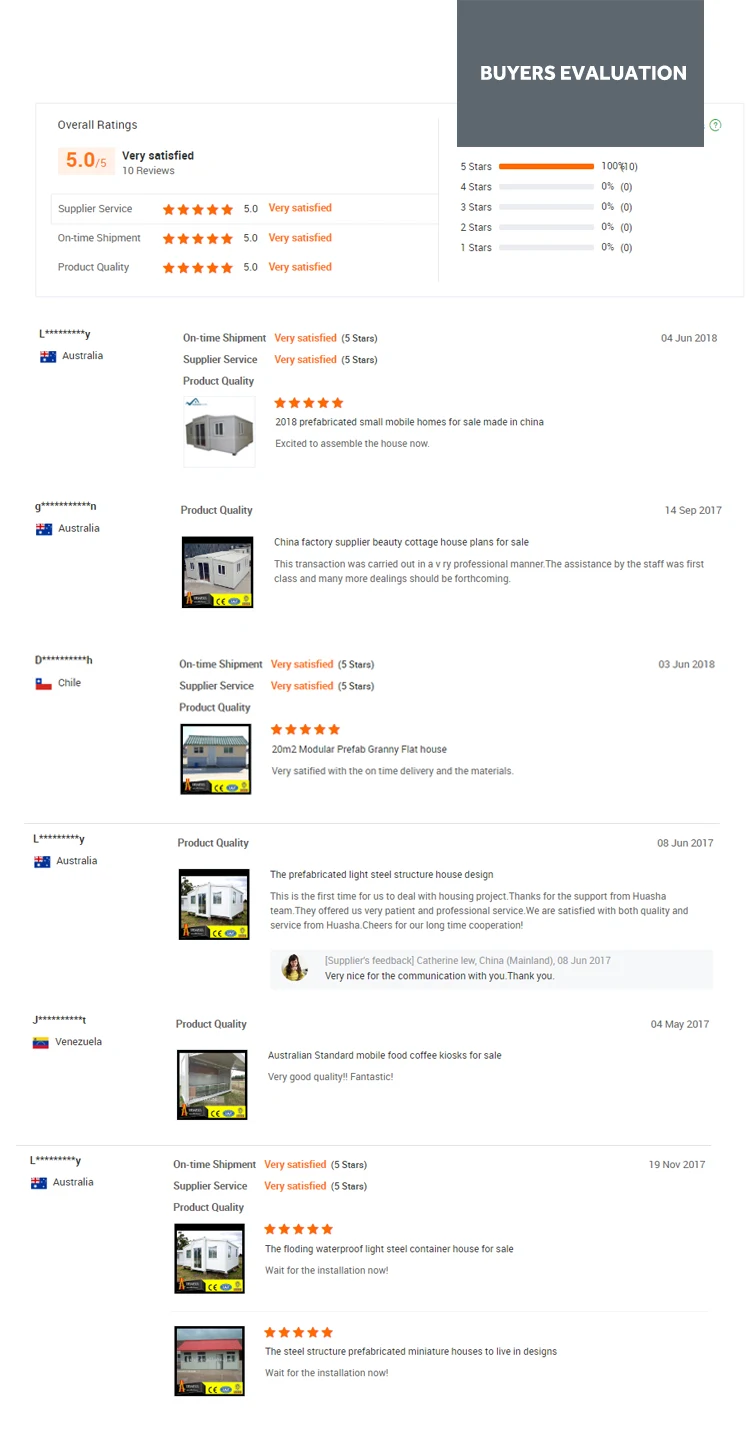In the image, the background is white, with a gray rectangle positioned in the top right corner. Within this rectangle, the text "Bias Evaluation" is prominently displayed in white. Underneath this section, a gray-outlined rectangular box is located, featuring several text elements detailing customer reviews and ratings.

On the left side of the box, the text "Overall Ratings" is displayed in black, followed by an orange rating of "5.0/5055." Below, in black, it signifies "Very Satisfied," mentioning that there are "10 reviews" providing feedback.

The next sections detail specific aspects of customer satisfaction:
- "Supplier Service: Very Satisfied"
- "On Time Shipment: Very Satisfied"
- "Product Quality: Very Satisfied"

The customer reviews specify different experiences and products:

1. From June 4th, 2018, one reviewer expressed excitement about assembling a "2018 prefabricated small mobile home for sale made in China," confirming their satisfaction with the on-time shipment.

2. On September 14th, 2017, another customer praised the factory supplier's "China, beauty cottage house plans for sale." This review highlighted the transaction's professional handling and exceptional staff assistance, anticipating more business dealings in the future.

3. A review from June 3rd, 2018, reiterated satisfaction with the on-time delivery and materials provided.

4. On November 19th, 2017, a customer commented on the "third and waterproof light steel container house for sale," noting they were awaiting installation.

5. Another review emphasized the "steel structure, prefabricated miniature houses to live in designs," describing the product quality as very good and fantastic.

This highly detailed and thorough feedback underscores the consistent satisfaction among customers with the product quality, on-time shipments, and supplier services.